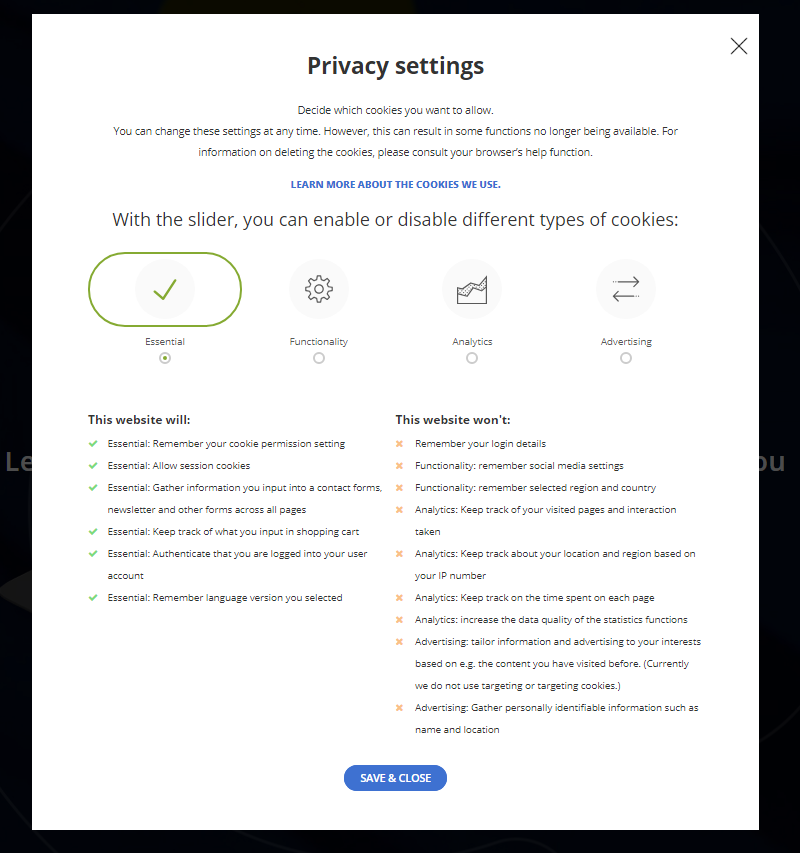This screenshot displays a privacy settings interface on what appears to be an 8.5 by 11-inch sheet of paper. The interface prompts the user to decide which cookies they want to allow. It explains that agreeing to these settings might result in some functions no longer being available. There is a recommendation to consult your browser for information on deleting cookies.

Below this explanation, there is a blue hyperlink labeled "Learn more about cookies," which users can click to obtain further information. The interface includes a slider mechanism that allows users to enable or disable different types of cookies. The slider is visually represented by a green-and-white circle with a green line around it.

Icons including a gear for general settings and an analytics icon are displayed next to navigational arrows pointing left and right. Below these icons, a section indicates that "This website will" followed by a list of supposed functionalities each with a green check mark, although the text is too small to read clearly. Another section states "This website won't" accompanied by twelve X marks, denoting functionalities that will be restricted.

At the bottom of the interface, there is a prominent blue button with white text that reads "Save and Close."